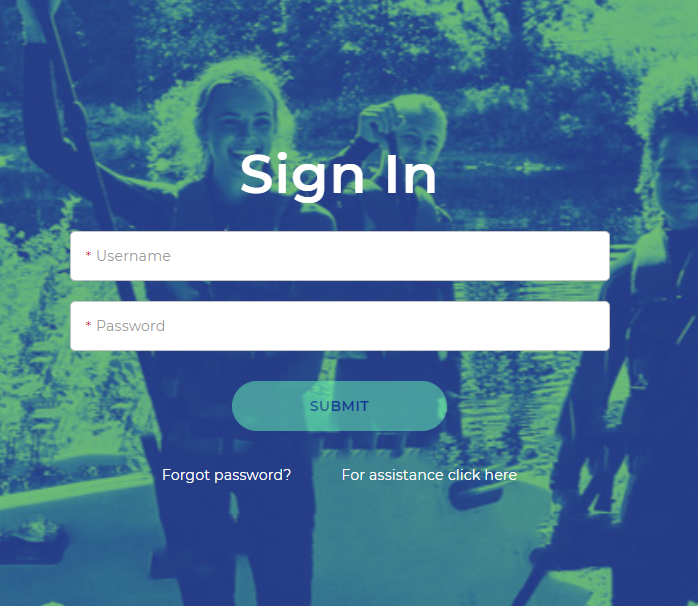The image appears to be a screenshot of a sign-in page on a computer. The background features an outdoor scene dominated by green and blue hues, showing three individuals engaged in what seems to be an outdoor activity. On the left, there is a female, while in the background and on the far right, there are two males. All three are dressed in black outfits and appear to be suspended by ropes, suggesting they are participating in a jumping or climbing activity among trees, visible in the center of the image.

The sign-in interface is overlaid on this background. At the top, in white text, it reads "Sign In." Below this, a large, narrow rectangle marked with a red asterisk is labeled "Username." A similar rectangle beneath it, also marked with a red asterisk, is labeled "Password." Following these fields, a green button labeled "Submit" invites users to proceed. Just under the submit button, in white text on the left, the phrase "Forgot password?" is displayed. To its right, also in white, reads "For assistance, click here."

The overall design suggests it is a login page, possibly for a website related to outdoor activities or events.